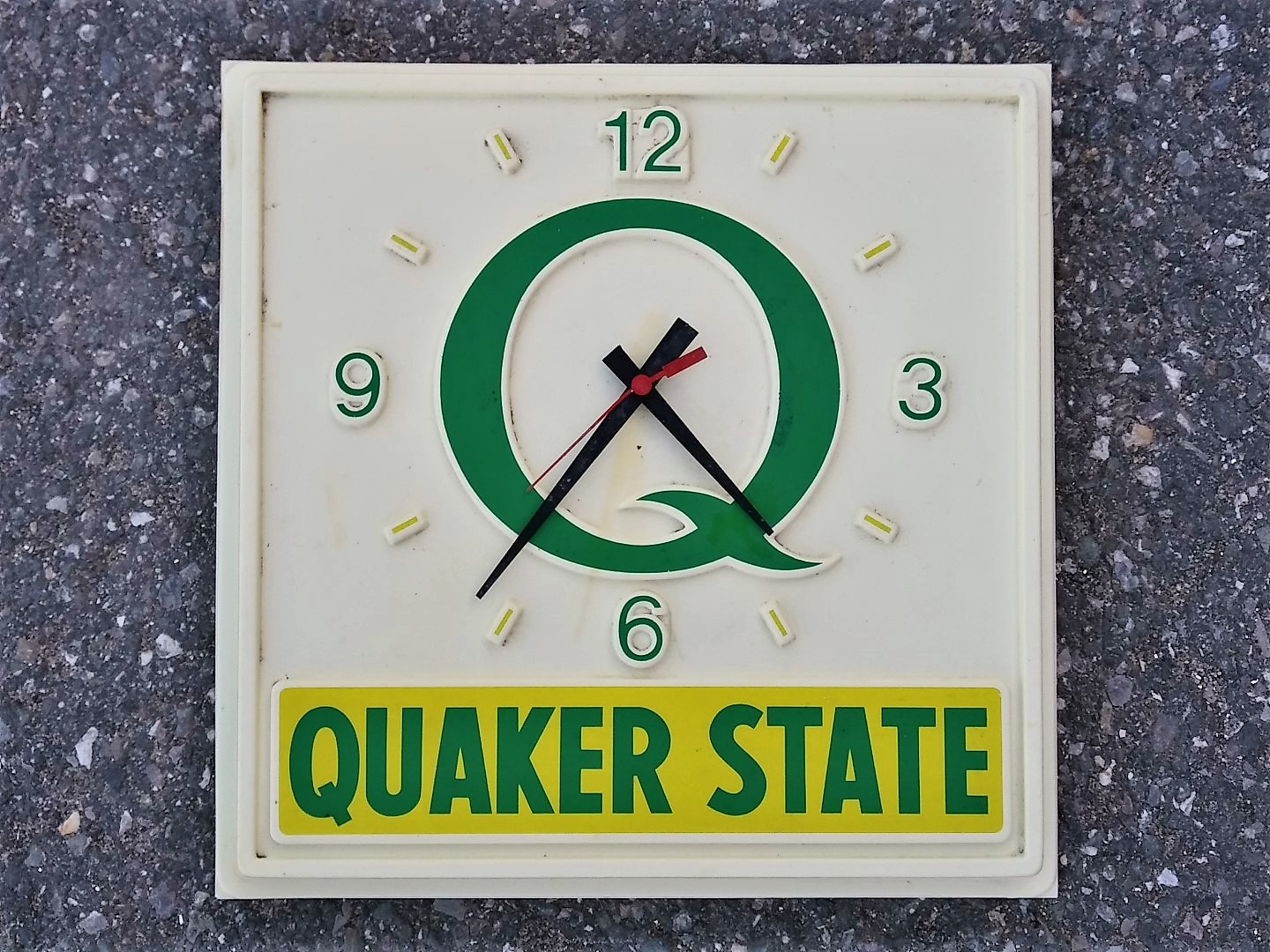The image depicts a vintage square clock with an off-white plastic frame, positioned against a dark gray surface speckled with white, brown, and lighter gray elements, possibly resembling a charcoal countertop or asphalt. At the bottom of the clock face is a yellow rectangular banner with "Quaker State" inscribed in dark green capital letters. Dominating the center is a large green 'Q', with black hour and minute hands and a distinct red second hand anchored from its middle. The clock displays the time as approximately 4:35 or 4:37. The numerals 12, 3, 6, and 9 are green, while the positions for the other numbers are indicated by white ovals with green centers. Moreover, small tick marks are present around the dial to denote minutes and seconds.